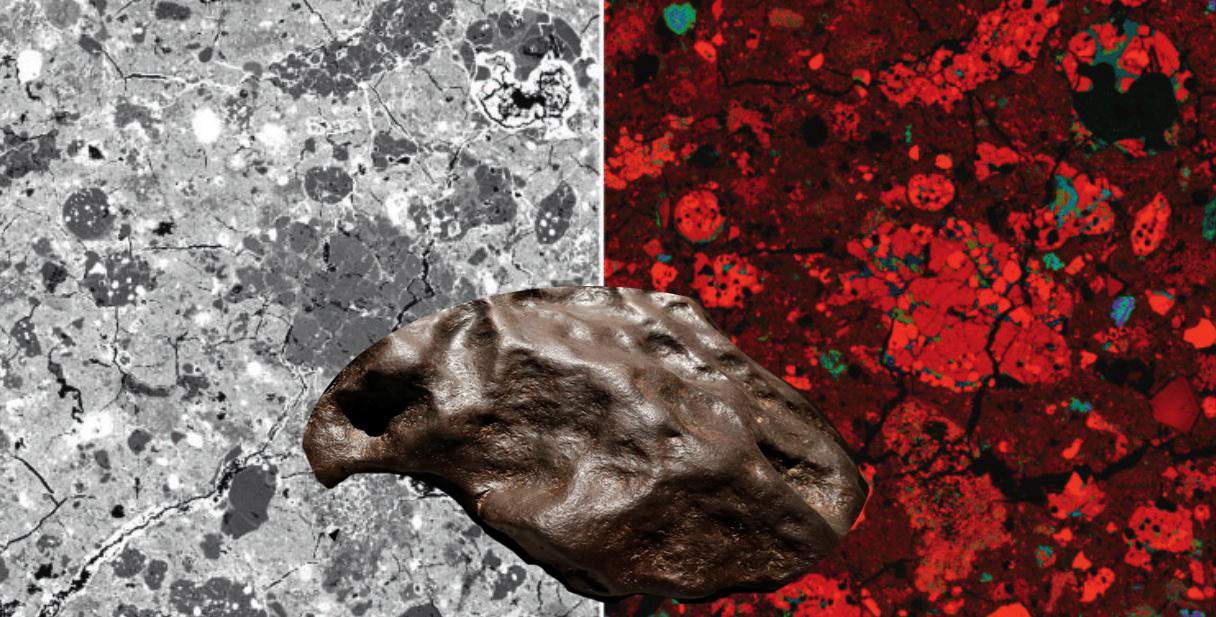The horizontally-oriented image features a split background composed of two square segments. On the left, the square displays a black, white, and gray marbled pattern with splotches and cracks, resembling a coarse, concrete-like texture. On the right, the square exhibits a dark red and light red marbled pattern, accented with subtle hues of green, blue, and teal, similar to a batik design. Together, these squares form a rectangle across the image. Centrally positioned at the bottom and spanning both squares is a peculiar, oblong, brown rock or sculpture. This object is characterized by its lumpy texture, multiple dents, and depressions, giving it an irregular, almost beak-like shape. The rock appears three-dimensional, as if it is placed on top of the marbled background. The image contains no text or additional elements.